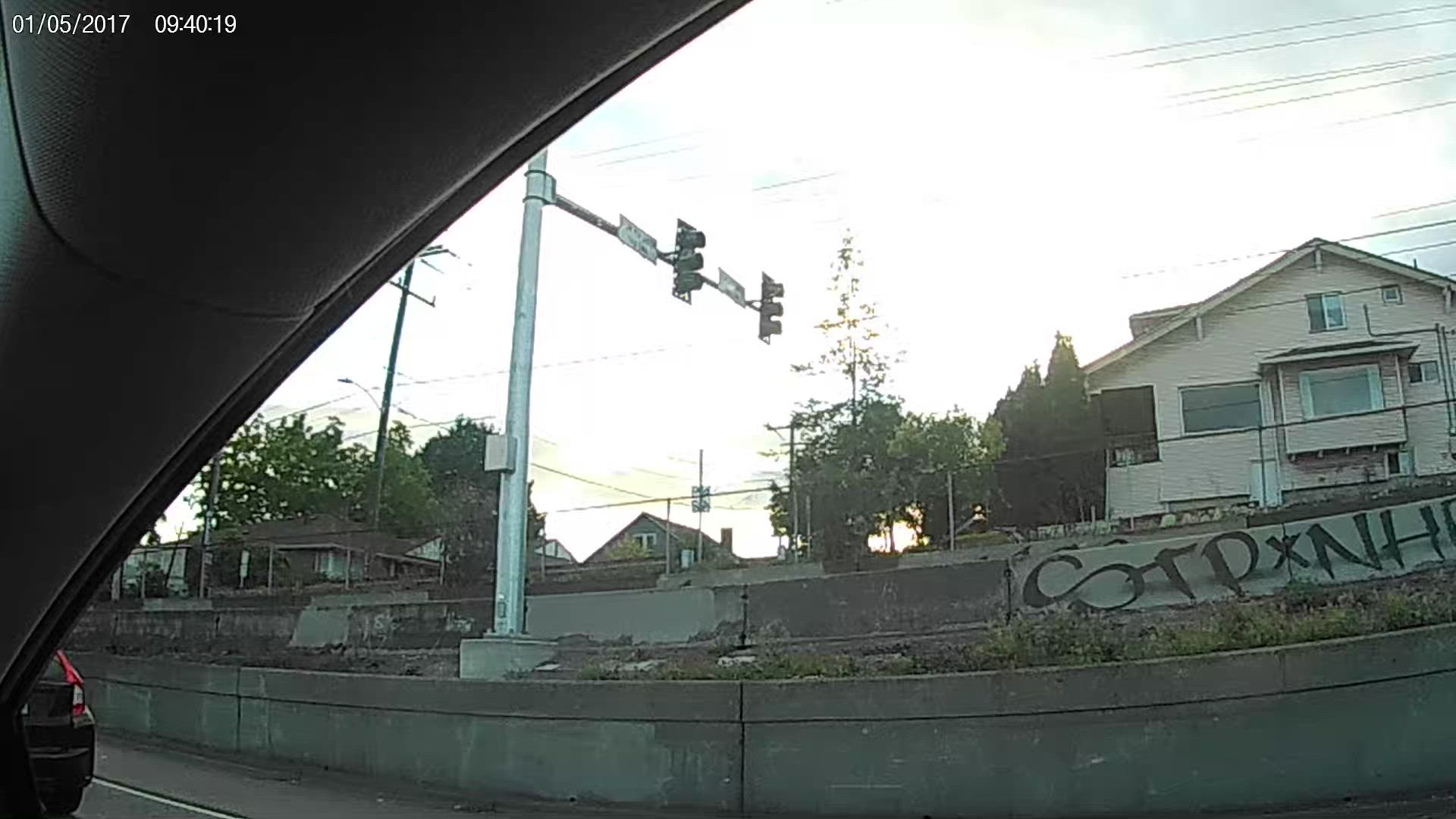This detailed photograph, taken from inside a car on a road or highway, captures the scene outside the front passenger window. Visible in the photo's foreground is a portion of the car's interior on the left-hand side, with a small black car alongside. A timestamp in the upper left corner reads "01-05-2017 09:40:19."

In the background, a concrete wall lines the side of the road, adorned with graffiti that partially reads "C-O-T-P-X-N-H," and separates the road from a hill. Atop this hill, a chain-link fence runs parallel to the road, beyond which three houses are visible. The closest house, buff-colored and slightly elevated on the hill, catches the eye first. To the left of this house and further back, a pink A-frame house comes into view, adding a pop of color to the scene. Partially visible between these two houses are segments of a third house.

Trees and bushes dot the landscape around the houses, while multiple stoplights and telephone poles with numerous lines crisscross the whitish sky above. The street scene is detailed with a traffic light mounted on a metal pole situated on a concrete curb, further enhancing the urban setting of this photograph.